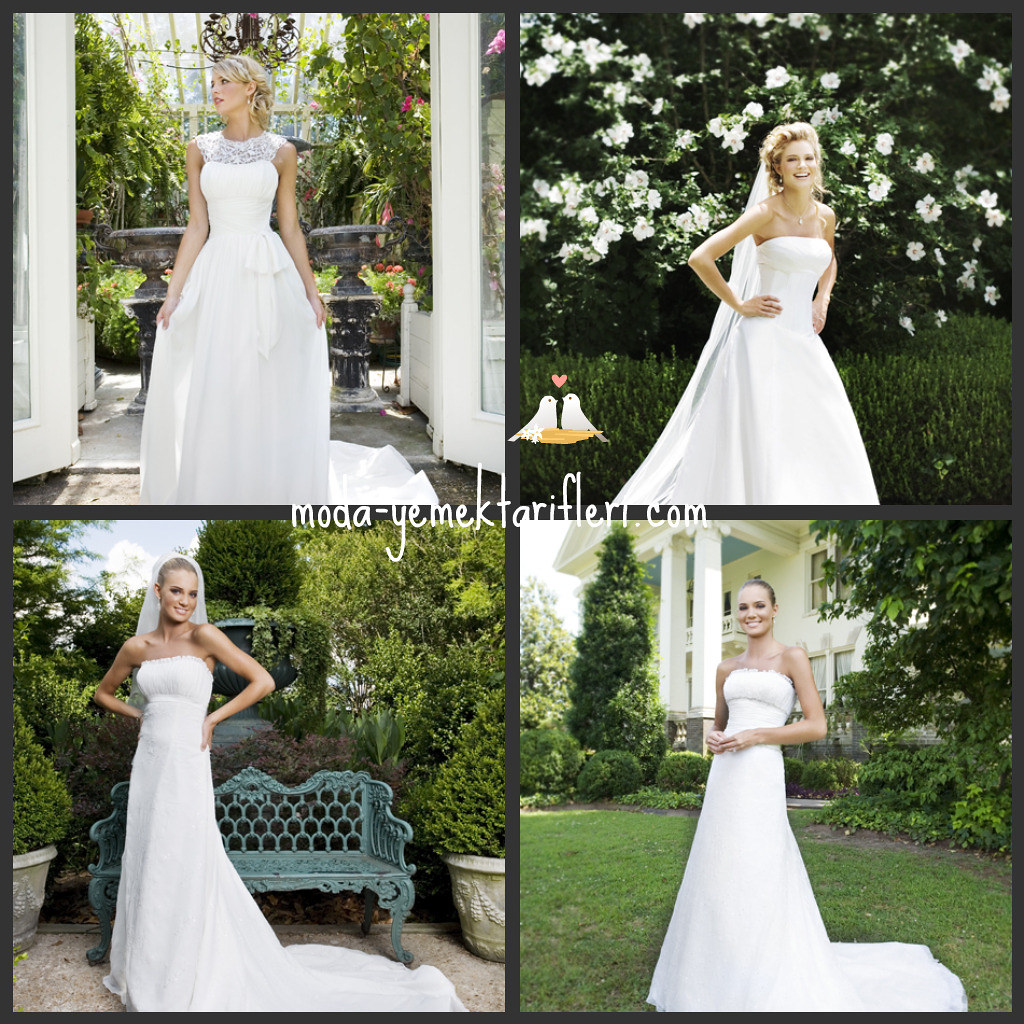This composite image features four photographs of a blonde model showcasing different wedding gowns, each set against various picturesque backdrops. The images are bordered by a thin black line and centered with the text "MODA-YEMEK-TARIFLERI.com" elegantly written in white script. 

In the upper left, the model wears a sleeveless gown with a lace bodice that wraps around her shoulders, standing gracefully before a greenhouse filled with lush flowers and plants. She holds the skirt wide, revealing the delicate pleats.

The upper right image depicts the same model in a strapless wedding dress. She has a long veil flowing behind her, though its attachment remains unseen. She poses in a yard in front of a vibrant bush adorned with white flowers. A charming cartoon of two white birds with a heart between them adds a whimsical touch to this scene.

On the lower left, the model dons the strapless gown again, complemented by a veil, as she stands beside a blue wrought iron bench set on a patio surrounded by greenery.

In the final image on the lower right, the model, now without her veil, showcases the strapless gown once more. She stands before a stately white mansion distinguished by its grand white pillars, neatly manicured lawn, and surrounding trees.